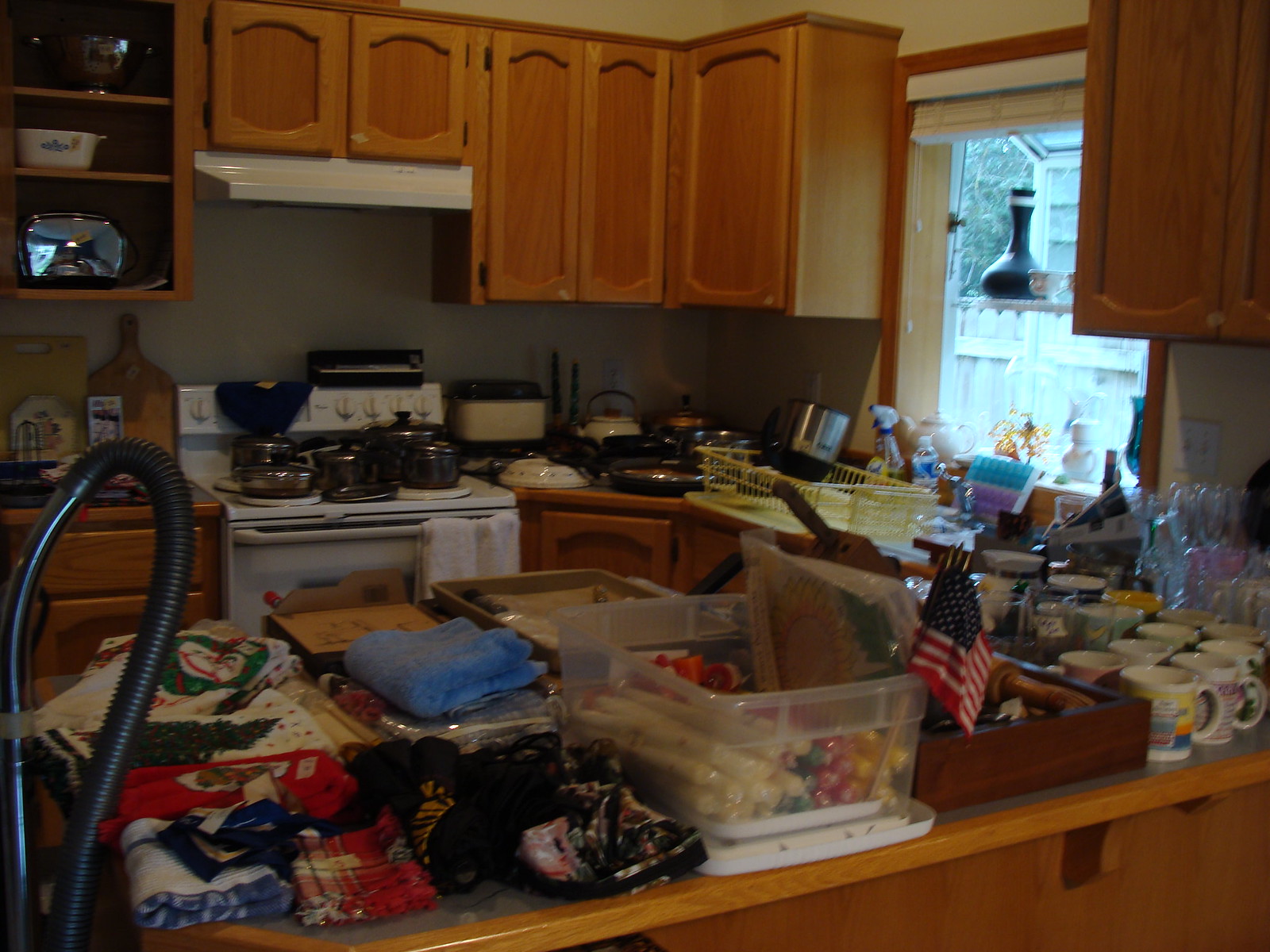The image depicts a bustling and cluttered kitchen with an array of items spread across the countertops. In the background, white kitchen cabinets and a stove with a range hood are visible. Several tea kettles in black and silver rest on the stove, accompanied by various pots and pans in silver and white. A window located in the right corner bathes the scene in natural light, revealing a glimpse of trees outside. On the windowsill, a black vase catches the eye. 

The sink in the foreground is filled with miscellaneous objects, while a blue dish towel lies nearby. To the left, a black vacuum cleaner hose is visible near two cutting boards, one dark wood with a handle and the other light wood with a groove for a handle. 

Closer to the front of the image, a heap of folded clothes in hues of red, blue, white, and green occupies a section of the countertop, alongside another folded blue towel. A transparent plastic storage bin, containing indistinguishable round objects, sits next to a small American flag. Nearby, a collection of teacups, primarily in gray and white, completes the scene.